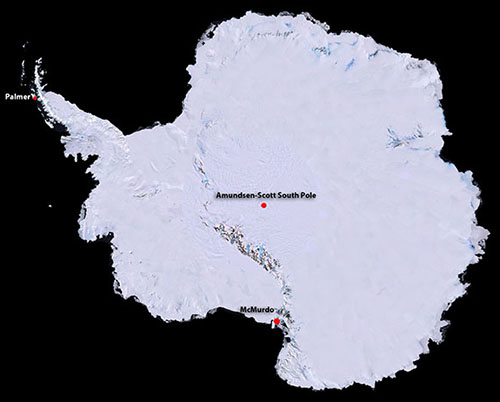This image features a detailed map view of the South Pole, showcasing a striking contrast between a black background and a bright white landmass, suggestive of a satellite view. The map displays three red dots indicating key locations: in the top left on a protruding section of the landmass is Palmer, centrally located in the middle labeled Amundsen-Scott South Pole, and at the bottom is McMurdo. The land's texture, possibly indicating mountain ranges or hills, is faintly visible, though the landscape predominantly appears whited out, focusing attention on the three labeled regions.